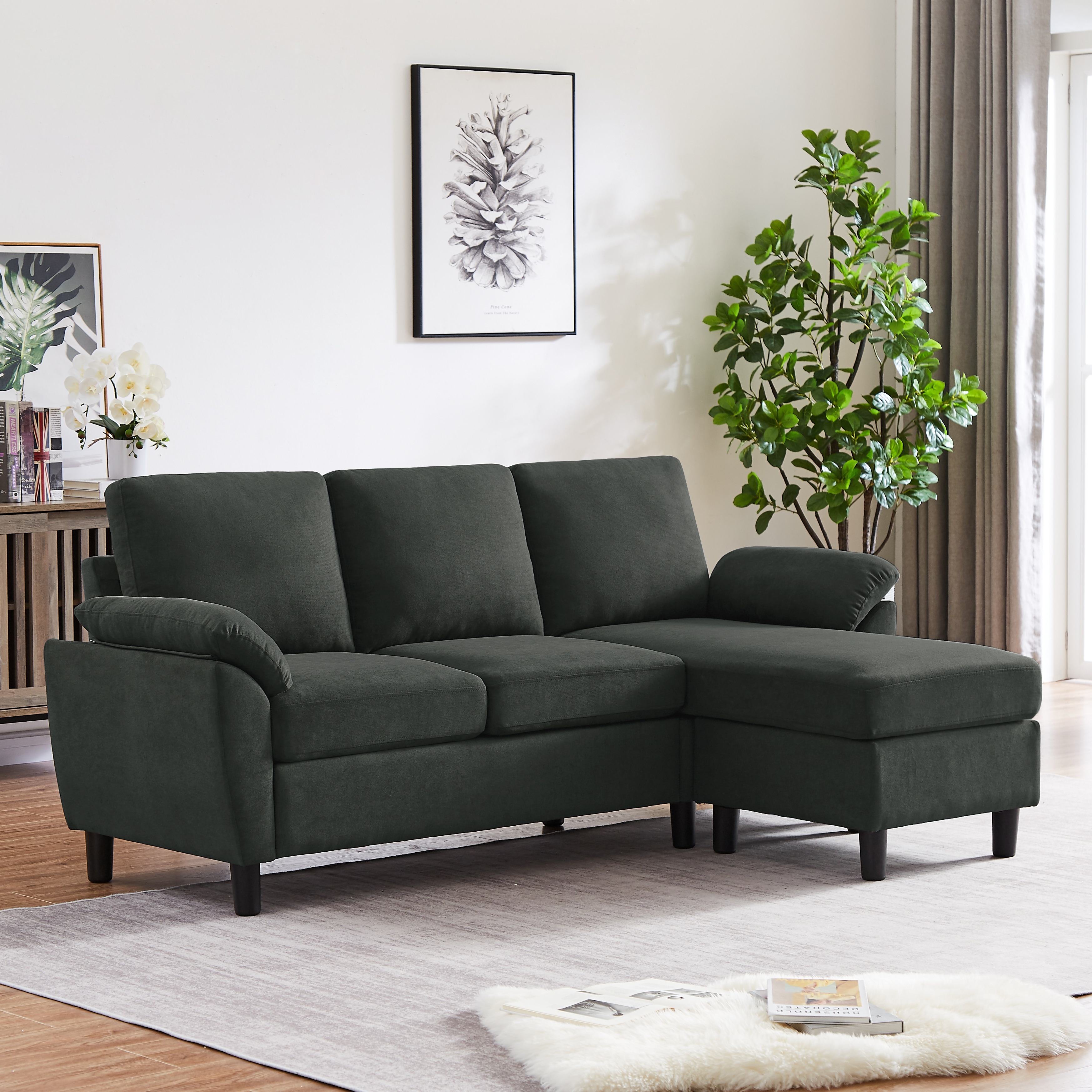This is a color photograph of a living room in a home, presented in a square format. The centerpiece is a dark gray suede sectional sofa with an L-shaped lounge extending to the right. The sofa has three large rectangular back cushions and three seat cushions, with the third on the right forming the chaise. Its short black legs jut out beneath its frame, and small pillows adorn each armrest. The sofa sits atop a wooden floor, partially covered by a large gray area rug with beige stripes. In front of the sofa, on the right side, lies a white furry rug with a couple of books and an open magazine scattered on it.

The background features a white-painted wall with a framed black-and-white print of a pine cone. On the right side of the image, a window lets in sunlight, highlighted by floor-to-ceiling beige drapes. Standing beside the drapes is an artificial green tree, partially concealed by the sofa. To the left of the image is a light-colored wooden sideboard topped with a vase of white roses and a few books. A framed picture of a fern leans against the wall above the sideboard, completing the cozy yet elegant decor.